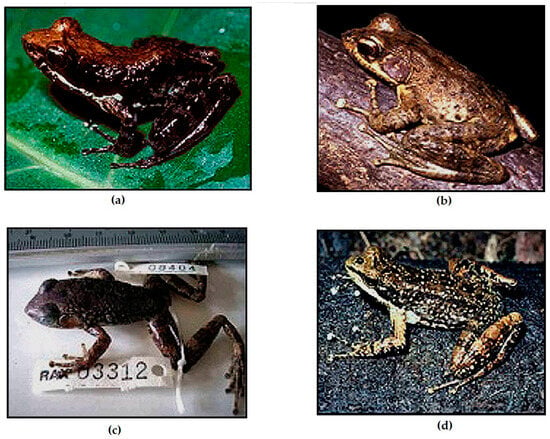The image features a series of four small photographs of frogs, each labeled A, B, C, and D, set within individual rectangles outlined by thin black lines and separated by white space. 

- **A:** A dark black and reddish-brown frog perched on a green leaf. This frog appears unhealthy with visible signs of distress.
- **B:** A muddy brown and tan-colored frog resting on a branch. Its earthy tones blend with the surrounding environment.
- **C:** A skinnier, dark brown frog that has a skeletal appearance, likely photographed in a lab setting, indicated by a ruler and tags nearby.
- **D:** A black frog with brown speckles, showing patches of yellow and white over its body, situated on soil. This frog also appears to suffer from some ailment.

Overall, the frogs manifest various disturbing conditions, suggesting they are not in the best of health. The image captures the diversity in frog species while also hinting at their environmental or health challenges.